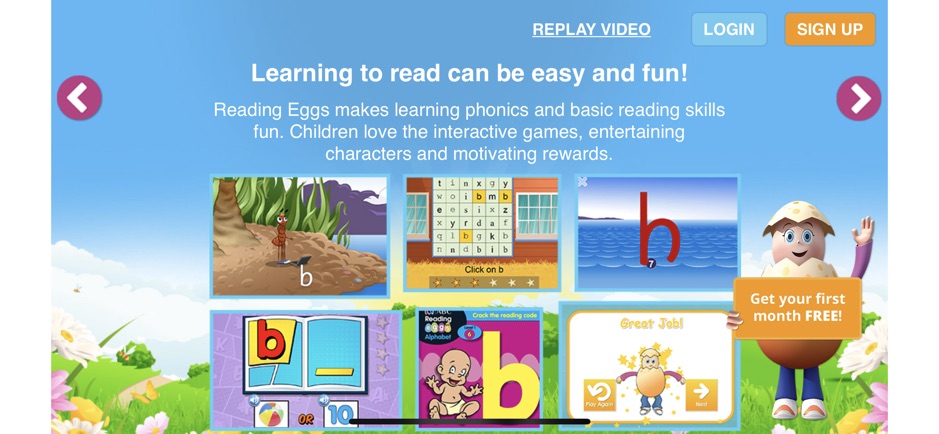The image features a vibrant blue background with various interactive elements promoting a fun and engaging reading program for children. At the top, it displays buttons for "Replay Video," "Log In," and "Sign Up." The central message reads, "Learning to read can be easy and fun. Reading Eggs makes learning phonics and basic reading skills enjoyable. Children love the interactive games, entertaining characters, and motivating rewards."

The visual highlights include:
- A large letter "B" adorned with grass, resembling a beach scene.
- A crossword puzzle.
- An illustration of a bee in a whimsical red ocean.
- A book featuring a bold red letter "B."
- A baby situated next to a letter "B."
- An egg icon with a refresh button on the left and a forward arrow on the right, promoting a first month free offer.

Additional elements include an egg character with expressive hands, face, and legs, accompanied by the text "Get your first month free." The background features green grass, blue skies, and a striking white mountain, creating an inviting and playful atmosphere. The image also includes the URL for free English learning resources: www.engvid.com.